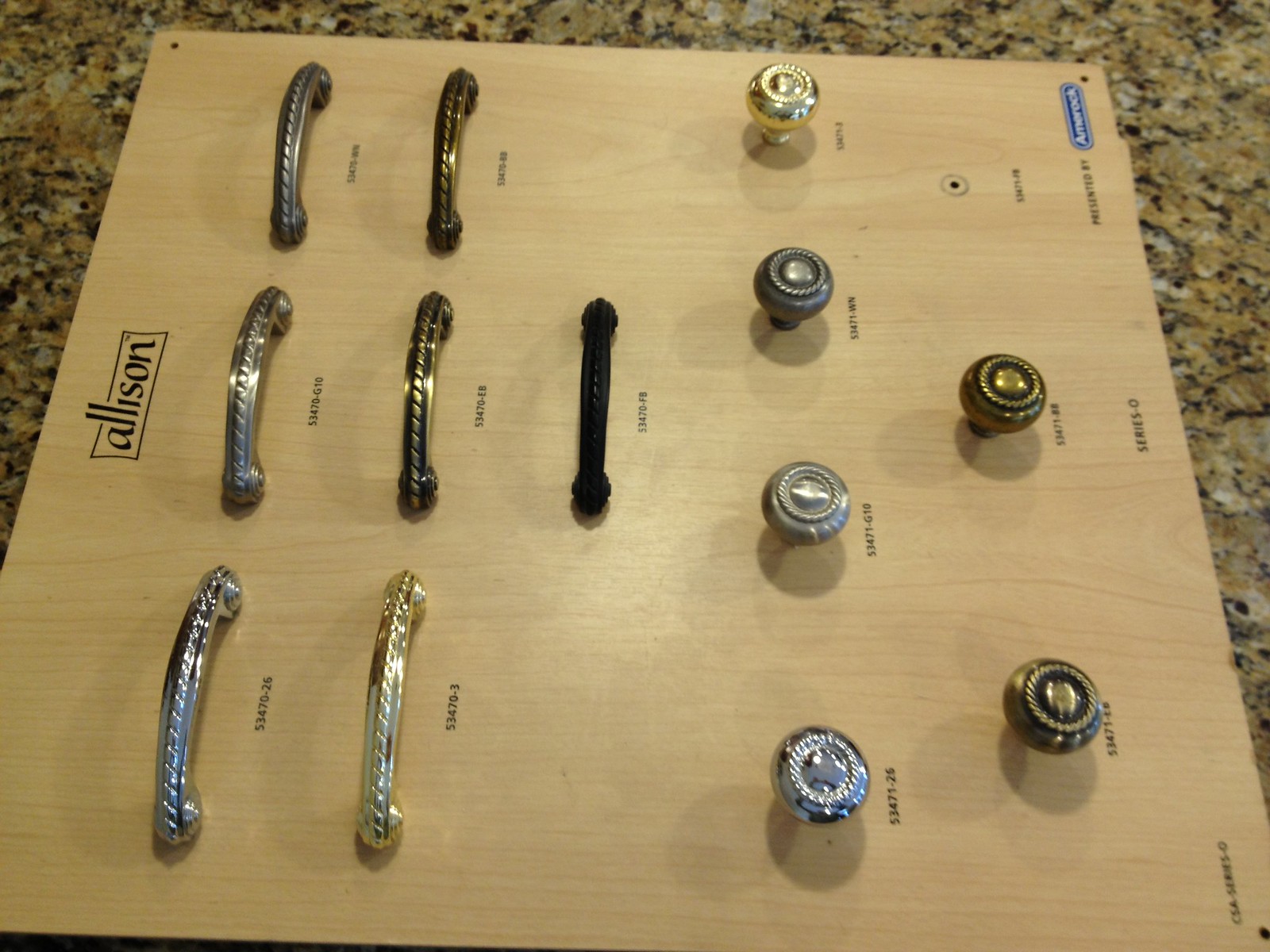The image depicts a detailed display panel that you might find in a store, set against a granite kitchen countertop that features brown, yellow, black, and white splotches. The display panel itself is made of light-colored brown wood, resembling bamboo. At the top of the panel, the name "Allison" is prominently displayed in black font, enclosed within a black rectangular outline. Arranged below the name are various metal drawer pulls and knobs, featuring a range of finishes including silver, gold, bronze, antique brass, and black. The pulls are organized in the upper section and are mirrored by corresponding knobs below them in the same metal finishes, though the black knob appears to be missing. These knobs and pulls exhibit different textures and patinas, from shiny to matte, enhancing their decorative appeal. In the bottom right corner of the panel, there is a blue rectangle with rounded edges containing text in white font, which is unfortunately too blurry to read.